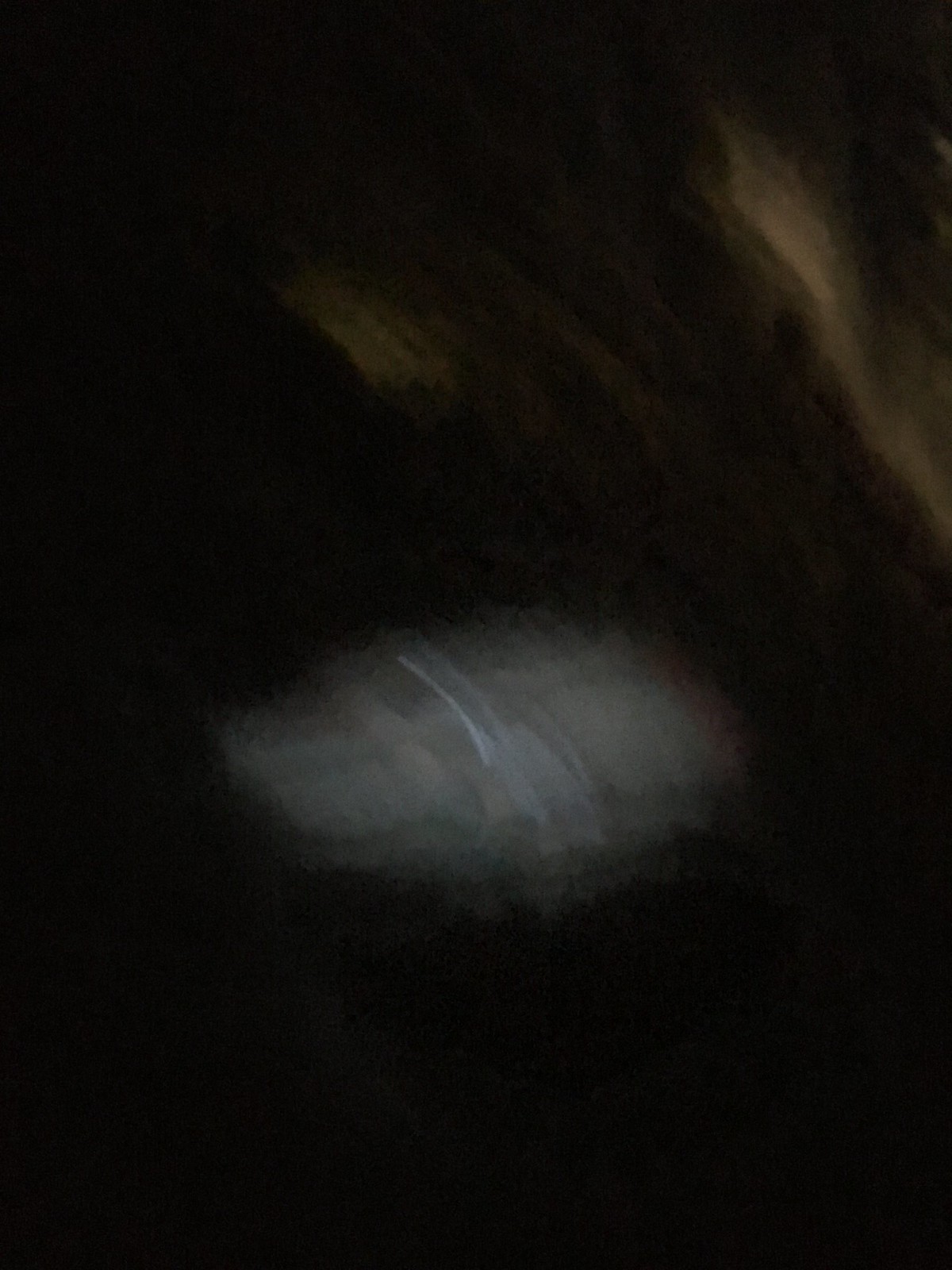This color photograph, taken in low light, is an abstract, heavily blurred, and virtually indecipherable image. The predominant background is solid black, suggesting it was taken at night. Central to the image is a rough, oval-shaped artifact, predominantly gray with hints of light brown and white tones, but its edges are undefined due to the blur. Above this central shape, approximately 60% down the image, there might be another abstract form resembling a squared-off mask, with a wide chin and forehead, appearing almost like it's made of cloud or smoke. In the upper right corner, there are diagonal streaks of light brown, which could be misinterpreted as tree limbs or other elongated objects. Another brown splotch is located just left of the center in the upper portion of the image. The entire photograph lacks clarity, making it difficult to determine what it actually depicts beyond these general shapes and colors.